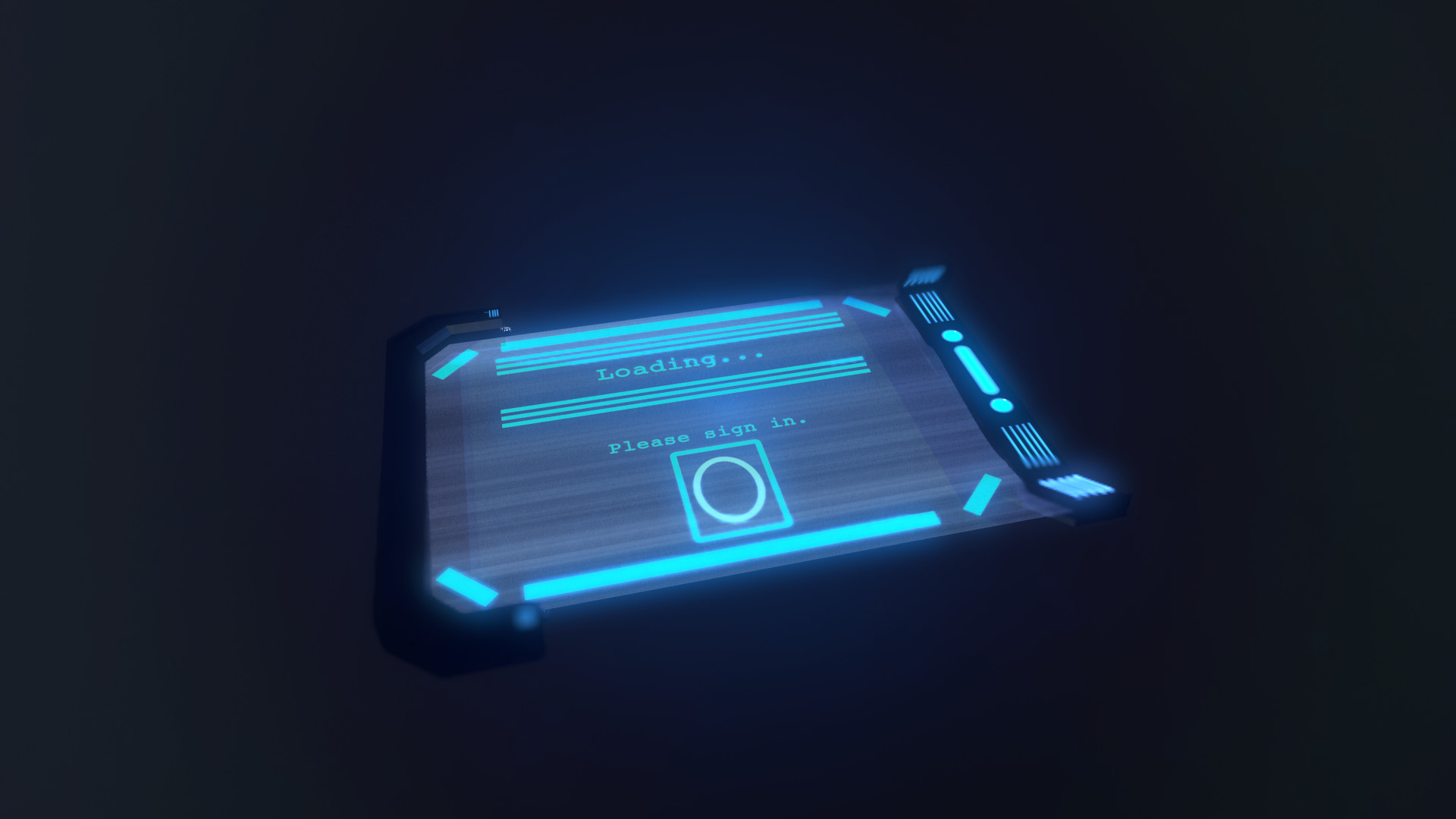In this image, a sleek, rectangular, round-cornered tablet or digital device is displayed against a pitch-black background. The device features black edges surrounding a primarily dark gray screen. Illuminated in vibrant blue light, the screen prominently displays the text "Loading..." followed by "Please Sign In." Above and below these phrases, horizontal blue lines add a design element, while at the very corners of the screen, additional horizontal blue lines can be seen. Centrally placed beneath the sign-in prompt is a vertical rectangle highlighted in blue, featuring a light gray button, presumably for user interaction to proceed with the sign-in process. On the right side of the screen, there are finer vertical lines and a thicker line topped with two circles, contributing further to the sophisticated, neon-blue digital aesthetic of the panel. The image is striking in its minimalism yet rich in digital design details, suggestive of a high-tech interface awaiting user engagement.